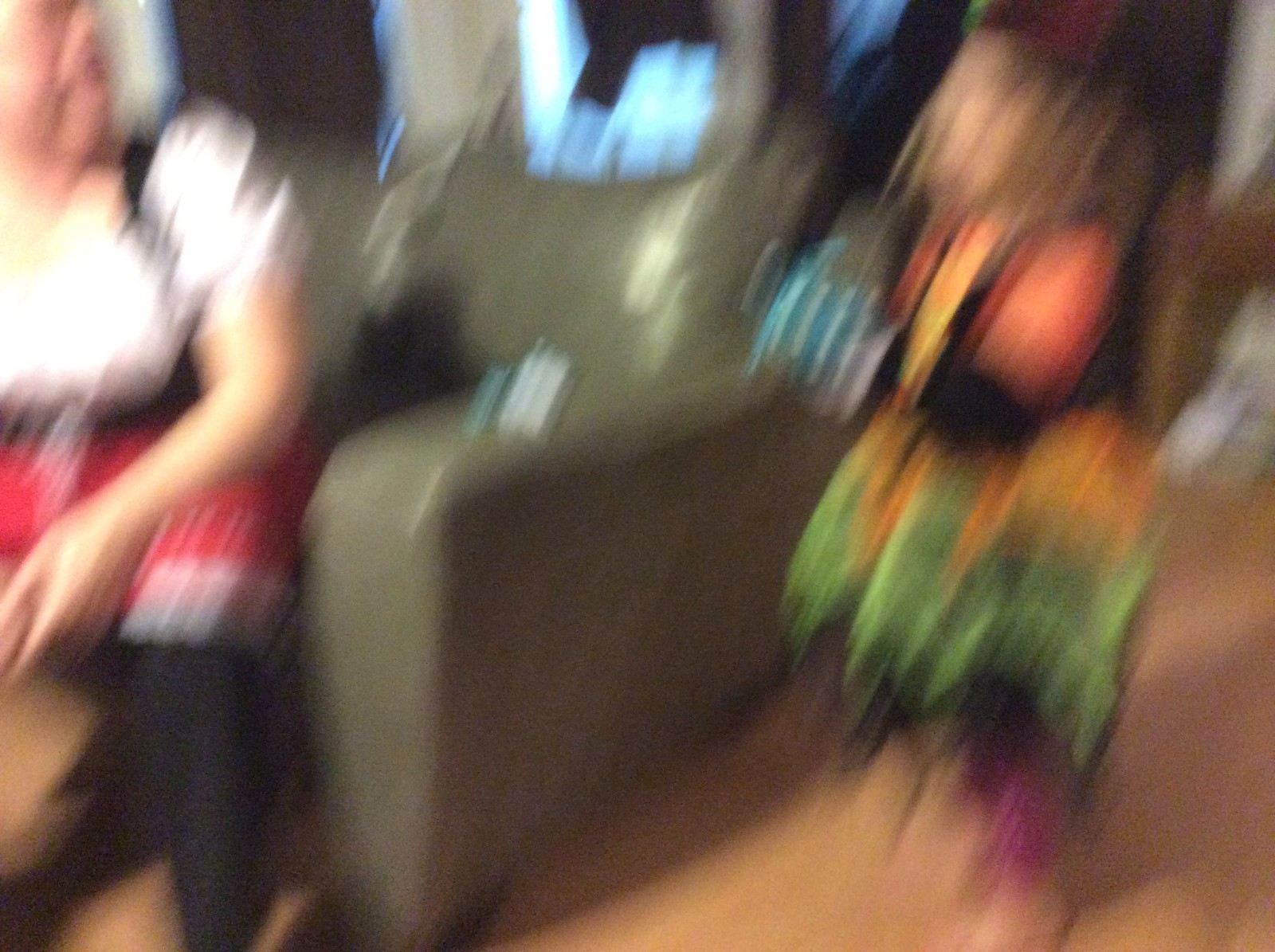The extremely blurry image appears to have been taken in a home, capturing a moment that seems linked to a Halloween event or an Oktoberfest-like gathering. In the foreground, there is a gray-green oversized couch or chair. Standing next to it is a child, likely a five-year-old girl given the context of Halloween, dressed in a vibrant and elaborate witch-like costume featuring colors such as green, orange, black, and purple. Her brown hair is either dark brown or a sandy color, possibly adorned with a bow, and she is holding something blue in her hand. 

Sitting beside her on the couch is an adult in a striking outfit that suggests they are dressed as a bar wench. The costume consists of a white top, red bottoms, and black stockings. The adult's gender is indiscernible due to the blurriness, but they complement the festive theme of the image. Additional details like the brown flooring and faint light in the back enhance the sense of an indoor setting during a celebratory occasion.